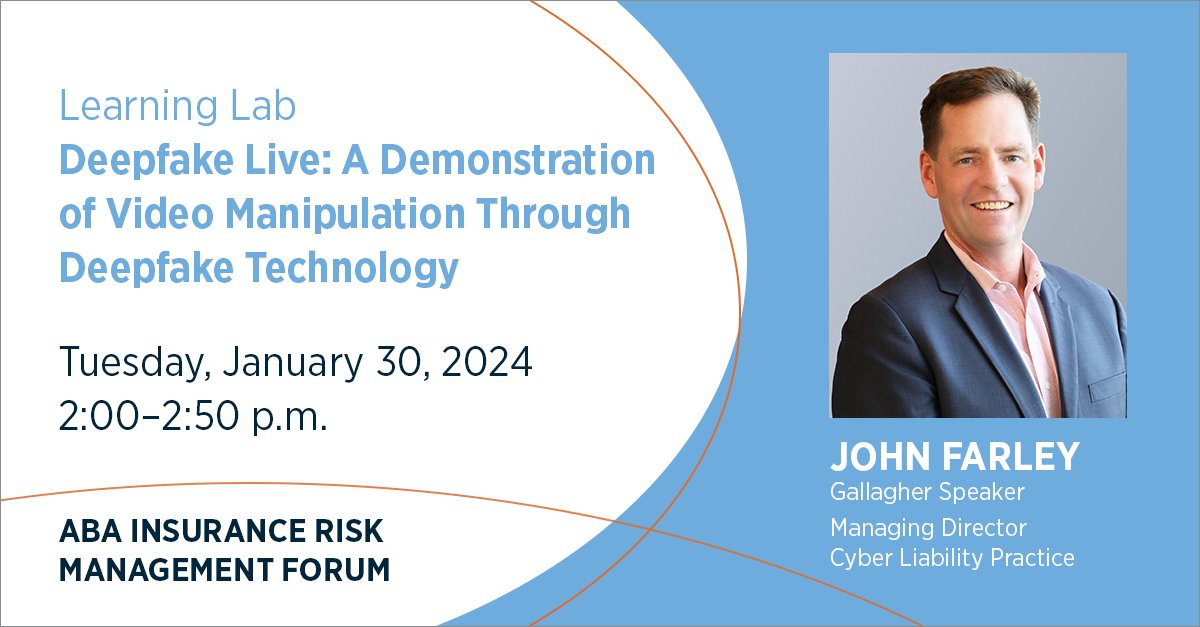The image is an announcement for the ABA Insurance Risk Management Forum, featuring a portrait of John Farley, a Caucasian man with short brown hair, dressed in a blue jacket and pink shirt. The announcement invites attendees to the "Learning Lab: Deepfake Live," a demonstration event showcasing video manipulation through deepfake technology. This event will take place on Tuesday, January 30th, 2024, from 2:00 to 2:50 p.m. John Farley is identified as a Gallagher Speaker and the Managing Director of Cyber Liability Practice. The layout of the announcement is divided, with the right side displaying John's photo and professional details, while the left side features the event information in blue and black lettering.